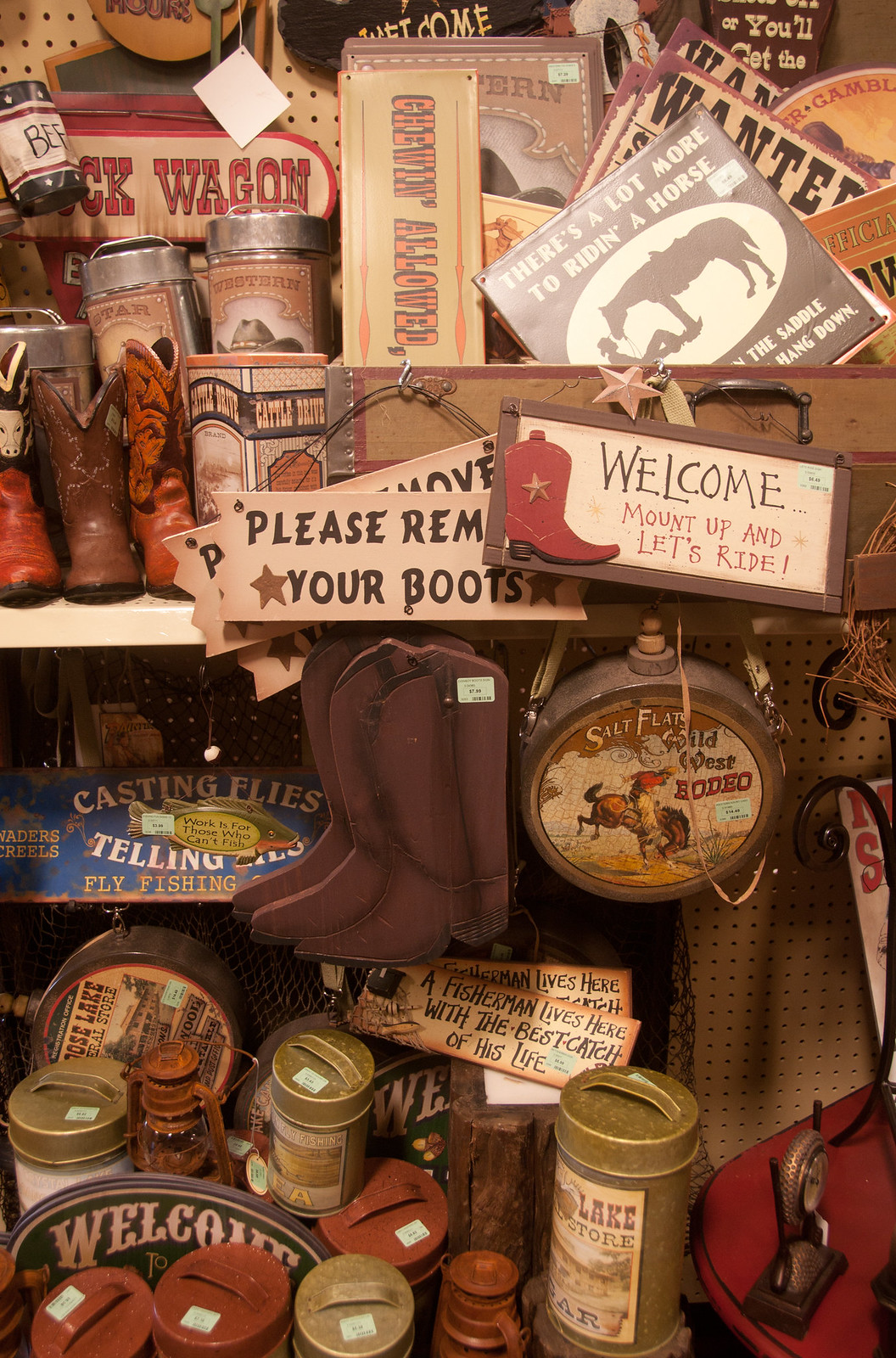The image captures a close-up view of a wall in a western-themed store, featuring a diverse array of antique and rustic items. Dominating the scene are various old metal cans, cowboy boots, and numerous signs, each brimming with charming slogans and phrases typical of the Wild West. The signs include messages such as "please remove your boots," "mount up and let's ride," and other playful prompts like "chewing aloud," and "fly-fishing." Some signs humorously declare, "a fisherman lives here with the best catch of his life." The wall itself has a tackboard appearance, with sections in the upper left corner showing a grid of holes where hooks might be inserted. The colors are predominantly earthy tones – beige, brown, and red – with occasional splashes of blue and metallic accents from tin cans. Adding to the ambiance are mounted sections for cowboy boots and other western paraphernalia. Overall, the image portrays a charming, cluttered snapshot of a nostalgic old-west gift shop or thrift store.